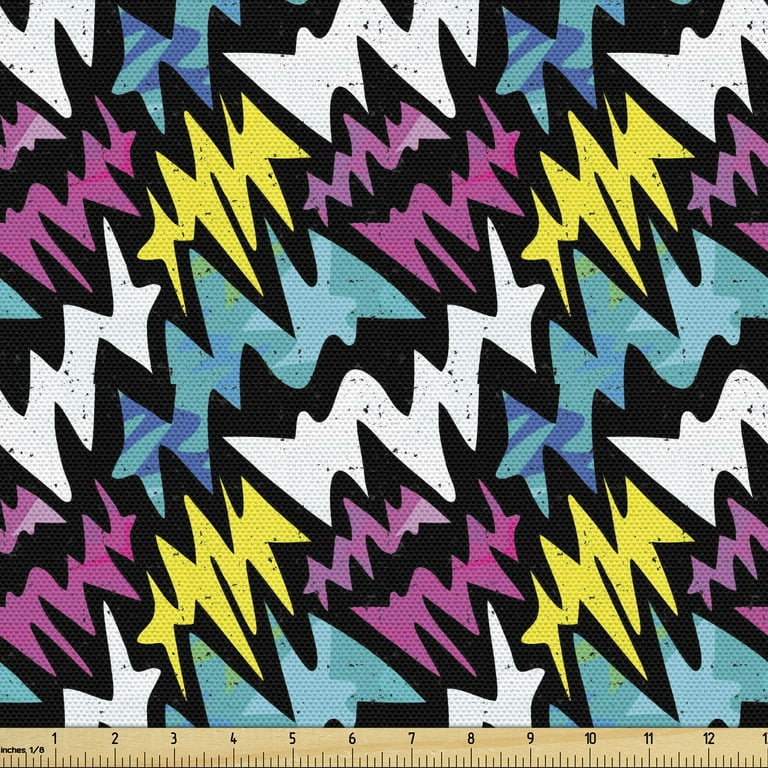The image is a vibrant and complex graphic design featuring an abstract assembly of squiggly lines and zigzags in various colors. Prominently displayed are lines in shades of yellow, purple, white, and multiple tints of blue including light blue, dark blue, sky blue, and turquoise. These lines, resembling thick lightning bolts or interconnected M shapes, are outlined in black and span diagonally across the poster. The intricate pattern includes approximately six white lines, four yellow lines, and six purple lines, all interwoven against a diverse blue background, which also contains teal and green hues. At the bottom of the poster, a wooden ruler is horizontally aligned, marked with black notches and numbers. The ruler, labeled "inches" at the starting point, displays measurements up to 13 inches, although only the '1' of the '13' is visible due to cropping. This combination of dynamic lines and the structured element of the ruler creates a visually engaging and busy design.